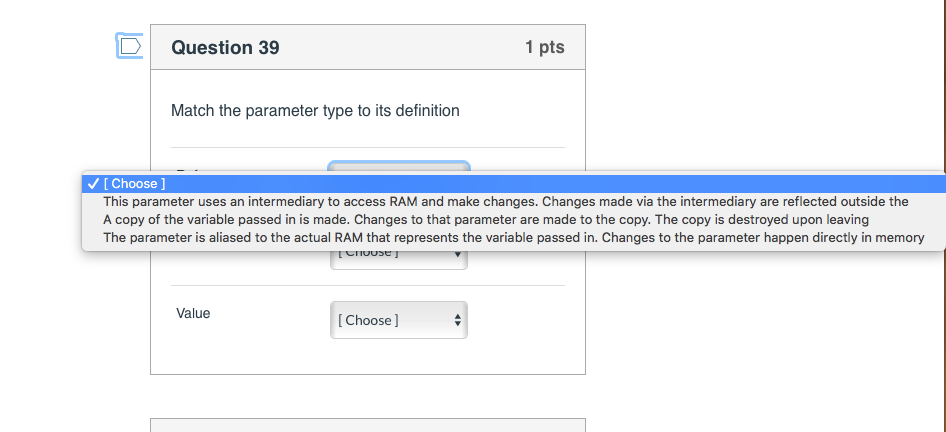This image captures a section of a larger website, likely an online test or quiz, designated as "Question 39" at the top. The question, worth one point, prompts users to "match the perimeter to the definition," indicating it may be part of an educational or assessment tool. 

Below the question header is a drop-down selection box for users to choose their answer. The question specifically inquires about the "value" and offers various definitions to choose from. A pop-up tool tip or help box extends beyond the boundaries of the main test content, presenting possible answers in blue-highlighted text.

The pop-up explanation details:
- "The perimeter uses an intermediary to access RAM and make changes. Changes made via the intermediary are reflected outside."
- "A copy of the variable passed in is made; changes to the perimeter are made to the copy, and the copy is destroyed upon leaving."
- "The perimeter is aliased to actual RAM that represents a variable passed in; changes in the perimeter happen directly in memory."

These statements seem to describe programming concepts related to memory management, such as pass-by-value and pass-by-reference mechanisms. 

Immediately beneath Question 39, another box is visible, indicating the beginning of Question 40, suggesting a continuous flow of questions in the test interface.